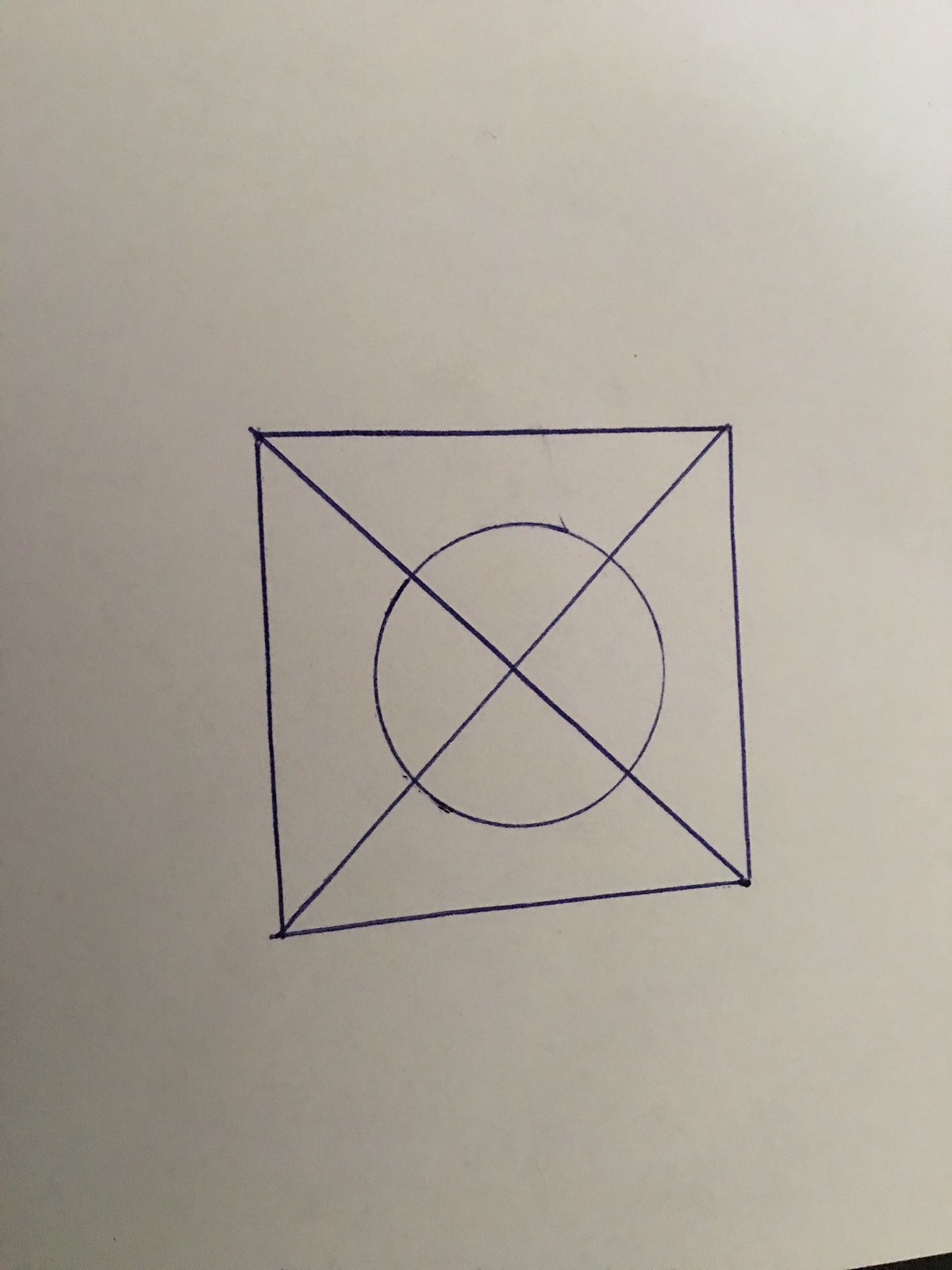The image depicts a sheet of paper with a diagram, slightly off-center toward the bottom of a pale grey background. In the bottom right-hand corner, a black bar is visible, possibly a frame or the surface on which the paper rests. The diagram features a square, tilted upwards to the right, creating a sense of imbalance. Drawn in black ink, the square is bisected diagonally from corner to corner by a line intersecting at the middle. From this intersection point, a not-quite-centered circle radiates, giving an uneven appearance potentially influenced by the paper's angle. Within the circle, small arrows suggest a direction of movement. The diagram appears incomplete, with no accompanying instructions to clarify its purpose.